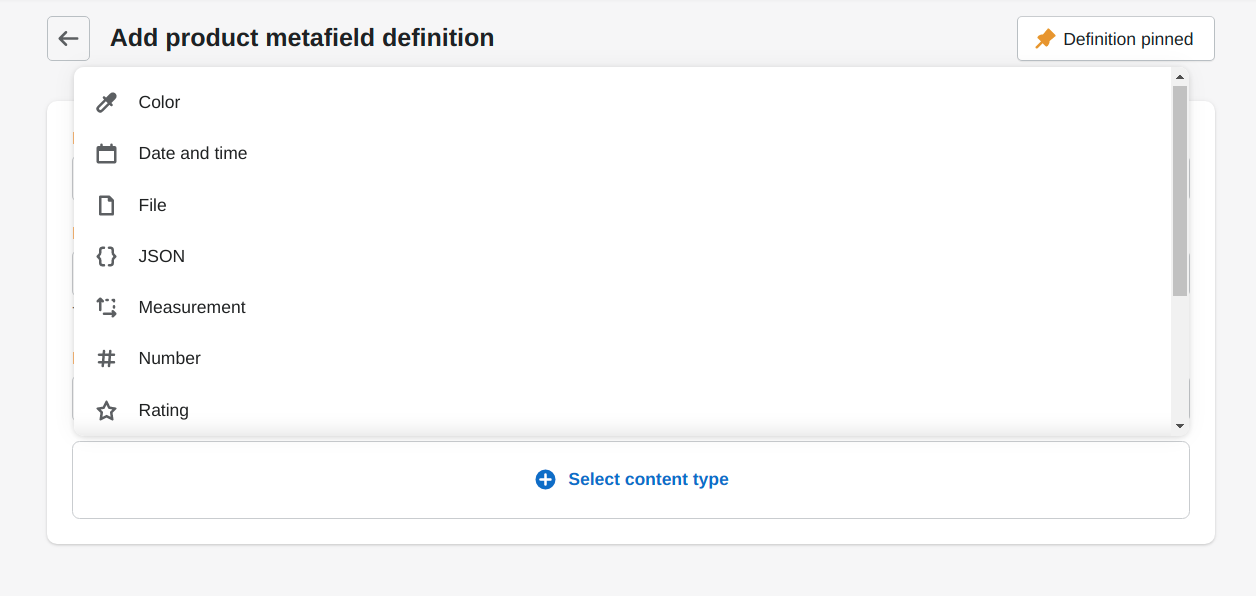The image depicts a settings interface for a program. The interface is framed by a large gray rectangular border, with a white inner section. At the top of this gray border, there is a text field that is labeled "Add Product Metafield Definition," indicative of the current task.

Below this text field, a dropdown menu is visible, featuring options such as "Color," "Date and Time," "File," "JSON," "Measurement," "Number," and "Rating." The dropdown menu can be scrolled further to reveal more options.

Centrally located on the interface is the text "Select Content Type," accompanied by a blue, link-styled plus sign enclosed in a circle, suggesting an actionable option.

In the top-right corner of the interface, there is a clickable box. On the left side of this box, a yellowish-orange thumbtack icon is present, followed by the text "Definition Pinned," indicating a pinned setting or definition. The overall design suggests a user-friendly and interactive environment for configuring product metafield definitions.